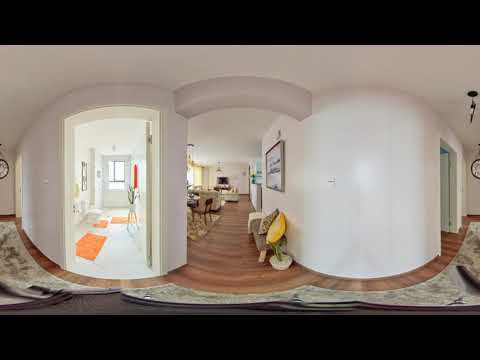The image depicts a detailed, panoramic view of a house with a modern yet classic and neutral design. The central area showcases a dining and living space with white walls and brown hardwood floors. At the center of the living area, there is a dining table with wooden chairs, a TV mounted on the wall, and a white sofa. A hallway leads into this space, featuring a bench adorned with a yellow pillow and a cheetah-print pillow. Additionally, several artworks and a clock embellish the walls.

To the left, there is access to a bathroom through a rounded entryway. The bathroom includes a window, a mirror, a toilet, and three orange or brown rugs. Right outside the bathroom, another clock is visible on the wall.

The right side of the image hints at a bedroom area, although it's not shown in detail. Another door in this area seems to lead to the kitchen. The overall aesthetic combines modern furniture and subtle, neutral tones, providing a warm and inviting atmosphere in someone's home.